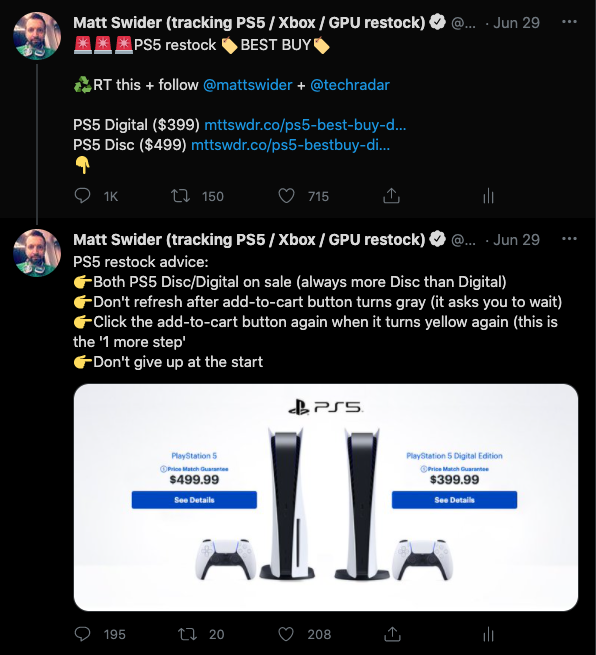The image is a screenshot of a Twitter feed, displayed on a solid black background. In the upper left corner, there is a small circular avatar featuring a man's face. Next to the avatar, in white text, it reads "Matt Swender" with a verification checkmark, followed by the description "tracking PS5 / Xbox / GPU restock" in parentheses. Below this text, there is a timestamp indicating the post was made on June 29th, as well as a three-dot options button.

The main body of the tweet includes three vibrant red icons related to the PS5 restock, with accompanying text stating "PS5 restock" and "Best Buy," surrounded by recognizable Best Buy logos. Directly beneath this, there is a recycle icon with the instruction "RT this + follow." It features a set of clickable Twitter channel links, labeled with "PS5 digital ($399)" and "PS5 disc ($499)."

A hand icon points downwards towards the typical Twitter interaction metrics, displaying the number of tweets, retweets, and likes. Below this section, there is a second entry from the same user, Matt Swender, with identical heading information.

This subsequent tweet, titled "PS5 restock advice," includes a list of four tips for securing a restock, each accompanied by a pointing right-hand icon. 

At the bottom of the screenshot, there is a prominent advertisement for the PS5, showcasing two purchase options: the PS5 Disc edition for $499 on the left and the PS5 Digital edition for $399 on the right. Both products are displayed alongside their respective controllers.